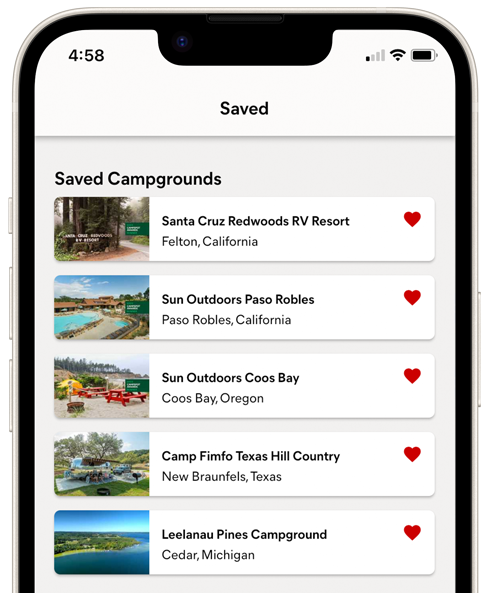The image depicts a black smartphone encased in a light gray or silver protective case. The visible portion of the phone occupies the upper three-quarters of the frame. The smartphone's screen displays a predominantly medium gray background, with the topmost section shaded light gray. 

In the upper left corner of the screen, the time is shown as 4:58 in black text, and to its right, icons indicate the battery is nearly full with a single signal bar. Across the light gray ribbon at the top, the word "saved" appears in black text.

Below the ribbon, information is organized into several horizontal white boxes. At the top of this list, in black text, it reads "Saved Campgrounds."

1. The first white box contains an image on the left depicting a forest trail. To the right, in black text, it reads "Santa Cruz Redwoods RV Resort, Felton, California," followed by a red heart symbol.

2. The second white box shows an image of a resort swimming pool. The text reads "Sun Outdoors Paso Robles," followed by "Paso Robles, California," with a red heart to the right.

3. The third white box features an image on the left of a campground scene with a picnic table, fire pit, and a tent. The text to the right reads "Sun Outdoors Coos Bay," with "Coos Bay, Oregon" underneath and another red heart to the right.

Additional entries are visible beneath these, continuing the list format.